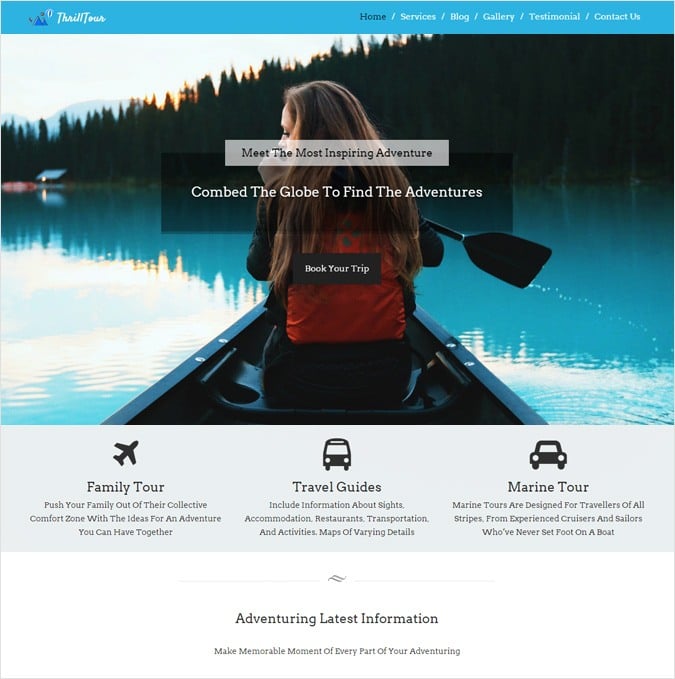This image showcases the homepage of the "Thrill Tours" website. 

On the left side of the banner at the top, there's a small icon depicting two mountains and a sun in dark blue. To the right of this icon, the website's name, "Thrill Tours," is elegantly written in white cursive lettering. Adjacent to the logo are the primary navigation buttons: Home, Services, Blog, Gallery, Testimonial, and Contact Us, all displayed in white font.

The background of the main section features an expansive landscape scene with a blue sky dotted with clouds. On the far left, part of a mountain peak is visible. Spanning the landscape are lush, tall trees, with a serene lake in the foreground. Central to the image, a woman is seen seated in a boat, paddle in hand. Captured from behind, her long brown hair cascades down her back, and her fair skin contrasts with the vibrant orange of her life vest. She appears to be looking to her left, adding a sense of curiosity and engagement to the scene.

Overlaying this picturesque background, a gray bar runs across the upper section with the text "Meet the most inspiring adventure" in bold black lettering. Below, another darker bar features the phrase "Comb the globe to find the adventures" in white text. Further down, positioned over the woman's life vest, the inscription "Book your trip" stands out in white.

Towards the lower section of the image, three categories are displayed: "Family Tour" on the left, "Travel Guides" in the center, and "Marine Tour" on the right, each indicating different offerings from Thrill Tours.